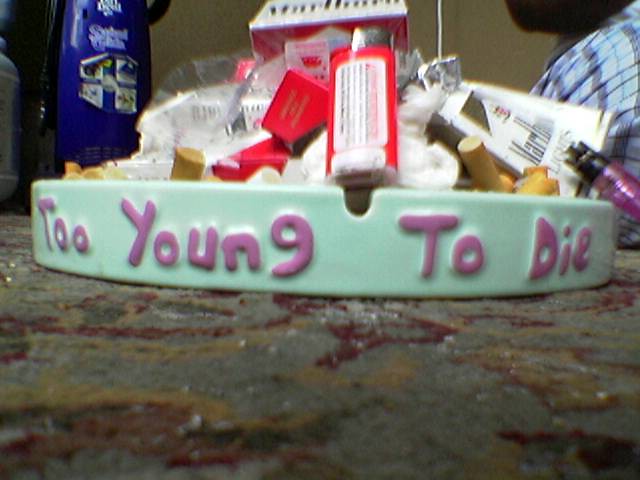The image captures a cluttered, ceramic ashtray prominently placed on a mixed-colored carpet, with shades of gray, burgundy, and gold. The ashtray, light green with pink embossed writing that reads "Too young to die," is filled to overflowing with smoking paraphernalia, including cigarette ends, discarded cigarette boxes—such as regular Marlboros and Marlboro Lights—pink and black lighters, and miscellaneous junk like a piece of foil and cotton. The setting appears informal and potentially outdoors, reminiscent of a pub garden or party scene. In the background, a hint of a person wearing a plaid cloth is visible, suggesting someone seated nearby, possibly next to a chair. Despite its chaotic content, the ashtray intriguingly looks like a hand-crafted project, adding a layer of irony to its state and inscription.